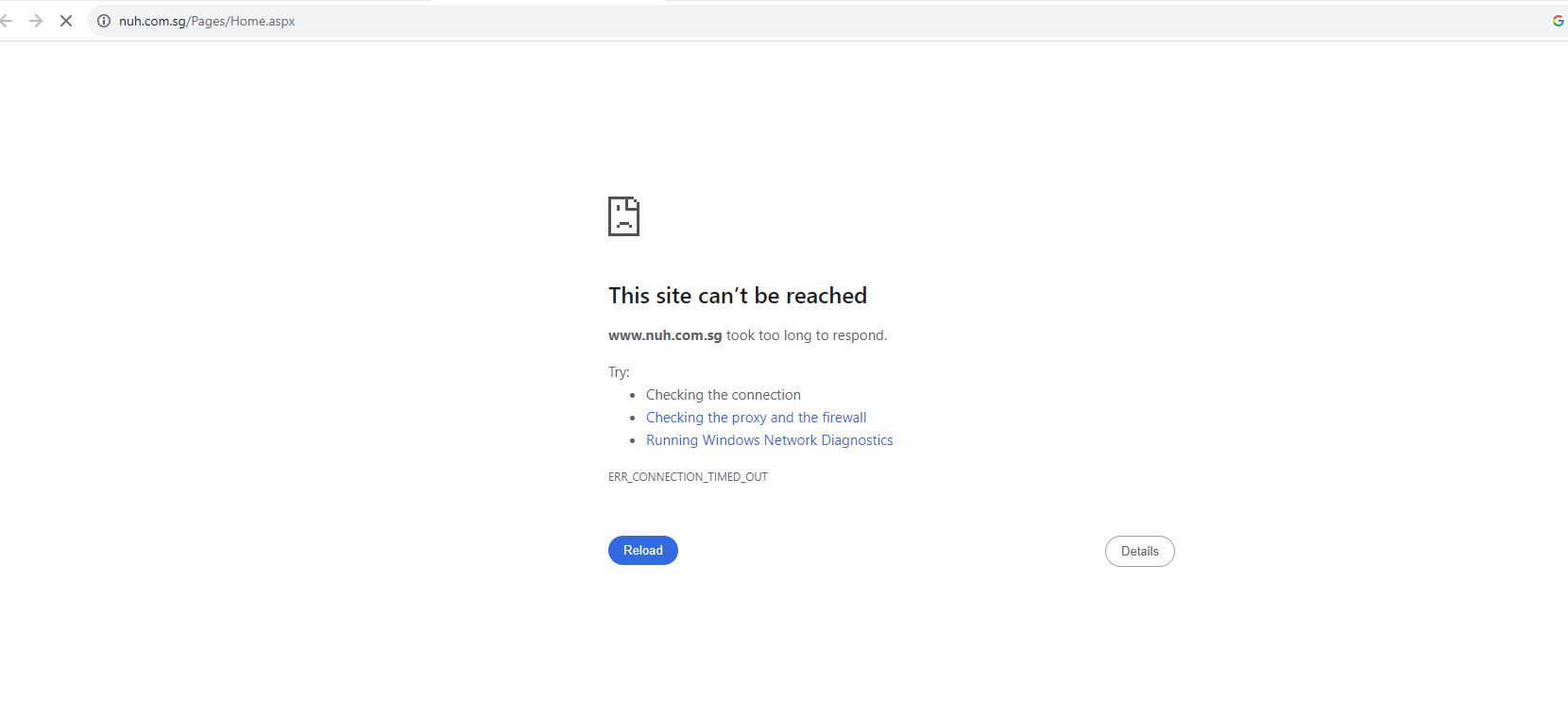The screenshot depicts a website page with a predominantly white header. At the far left of the header, there is a light gray arrow pointing left, followed by another light gray arrow pointing right. To their right, there is a dark gray "X". Next, a light gray URL bar with rounded corners contains a dark gray circular 'i' icon at its far left, followed by the URL "ne.com.sg/home.aspx" in black and light gray text respectively. On the far right of the URL bar is a multicolored 'G' icon. Beneath the header, a thin light gray line separates it from the body of the page, which is also white.

On the upper left of the body of the page, there is a dark gray icon depicting a piece of paper with its top right corner folded over, featuring an eye icon to its left and a frowny face beneath it. Directly below this icon, bolded black text reads, "This site can't be reached." Further down, left-justified dark gray bolded text shows the URL "www.ne.com.sg," followed by light gray text stating, "took too long to respond." Below, light gray text suggests three troubleshooting steps prefaced by "Try:" in dark gray. The first step, "Checking the proxy and the firewall," is listed in gray text, while the subsequent steps, "Running Windows Network Diagnostics" and another unspecified action, are in blue. At the very bottom of the page, in small all-caps light gray text, an error code reads, "ERR_CONNECTION_TIMED_OUT."